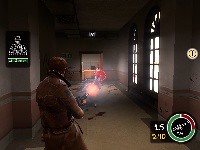The image appears to be from an action sequence in a Resident Evil or similar survival horror video game. Dominating the foreground is a character with short brown hair, clad in a brown leather jacket, actively firing a rifle. The rifle's muzzle flash is clearly visible in the image. Splashes of red, likely blood, are prominently scattered across the white floor, adding to the scene's intensity.

In the backdrop to the right, there's a closed door with a door rail, partially visible, suggesting an industrial or laboratory setting. Two other doors are open, allowing remnants of blasts—potentially from previous gunfire—to be seen. There are a total of eight blast marks visible, indicating a heavily contested area.

In the graphical overlay, the top left corner displays a black square with the outline of a person in white, accompanied by a green bar, possibly indicating the character’s health status. The bottom right corner shows a gauge resembling a radar or diagnostic tool, with segments in green and some in red, and a hand-like dial centered in the middle. To the left of this gauge, the number "1.5" is indicated, while a yellow element rests underneath. At the top right corner of the image, a white circle surrounded by blue, containing a fountain-like symbol, can be seen on a wall, suggesting an environmental clue or game mechanic.

Overall, the scene is grainy, lending it an old, retro aesthetic typical of earlier video games in the genre.